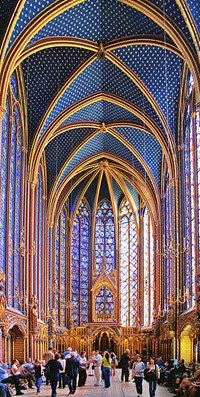The image depicts the interior of a grand cathedral with a strikingly tall ceiling that extends tens of feet high. The ceiling is highly elaborate, designed with triangular patterns in navy blue, adorned with white polka dots, and divided by curved gold outlines. Surrounding the space are immense, arch-shaped stained glass windows that stretch vertically, filling three visible walls with their intricate blue and white designs. The floor, likely made of marble, appears to be white, while various golden archways can be seen in the distance below the windows. The perspective of the image emphasizes the height and grandeur of the cathedral, making the people on the ground seem small in comparison. Groups of visitors are scattered on the floor, gazing up at the magnificent ceiling, immersed in the awe-inspiring atmosphere of this ornately detailed, historic building.